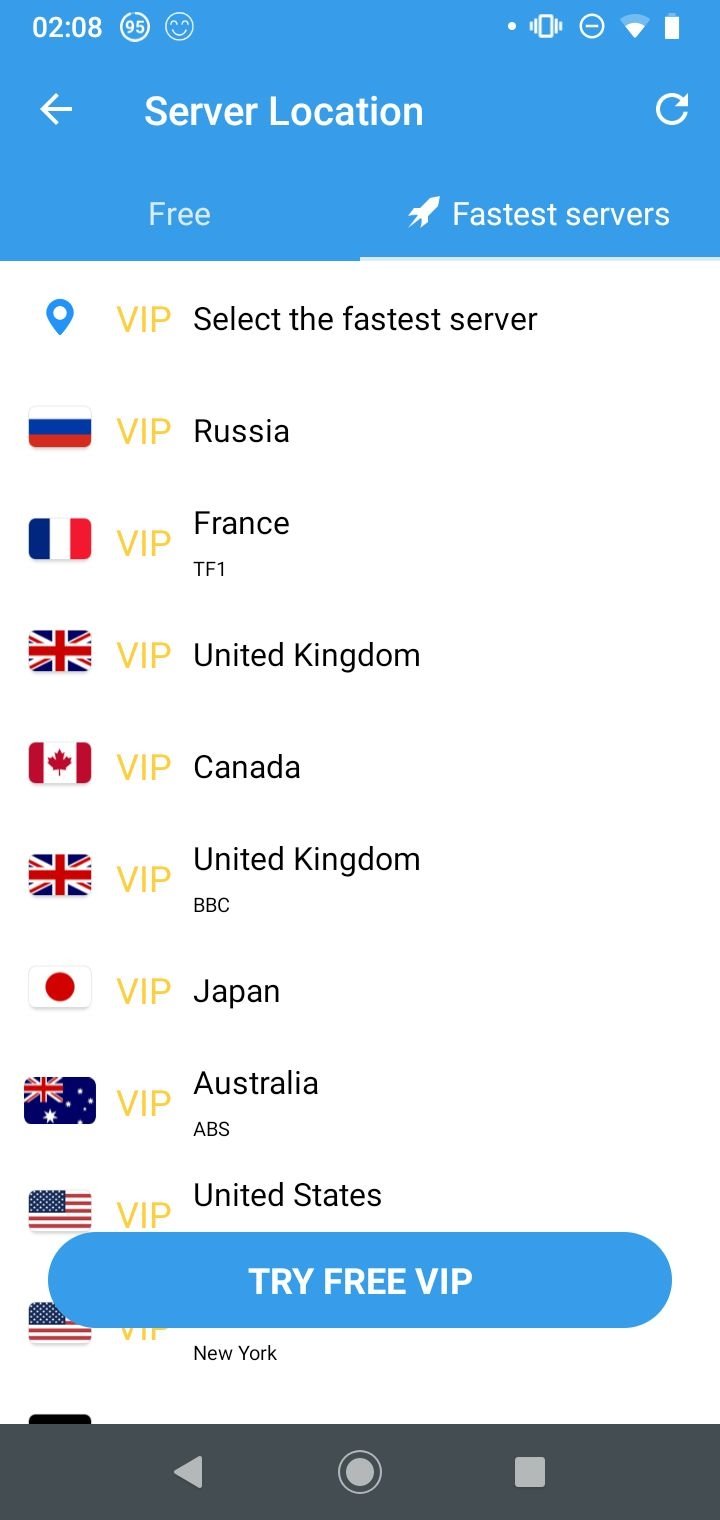This image is a screenshot of a VPN selection interface. 

At the top, there is a blue header bar displaying the time "2:08", along with some unidentified symbols towards the right corner. In the middle of this blue bar, there is an arrow pointing to the left labeled "server location" and to the right, there's a refresh button. At the bottom of the blue bar, it says "free" with a rocket ship icon next to it, followed by the words "fastest servers".

The main section of the screen is white, featuring a blue pin icon and the word "VIP". Below this, the text reads "select the fastest server". Listed are various server locations with country flags and VIP labels:
- The Russian flag, labeled "VIP Russia"
- The French flag, labeled "VIP France TF1"
- The UK flag, labeled "VIP United Kingdom"
- The Canadian flag, labeled "VIP Canada"
- Another UK flag, labeled "VIP United Kingdom BBC"
- The Japanese flag, labeled "VIP Japan"
- The Australian flag, labeled "VIP Australia ABS"
- The American flag, labeled "VIP United States"
- There's another selection with the American flag, unreadable due to an overlaying bar.

Below these options, it says "New York". There is a blue bar above this text that reads "try free VIP". Finally, at the bottom, there's a gray bar containing a back arrow, a dial button, and a square.